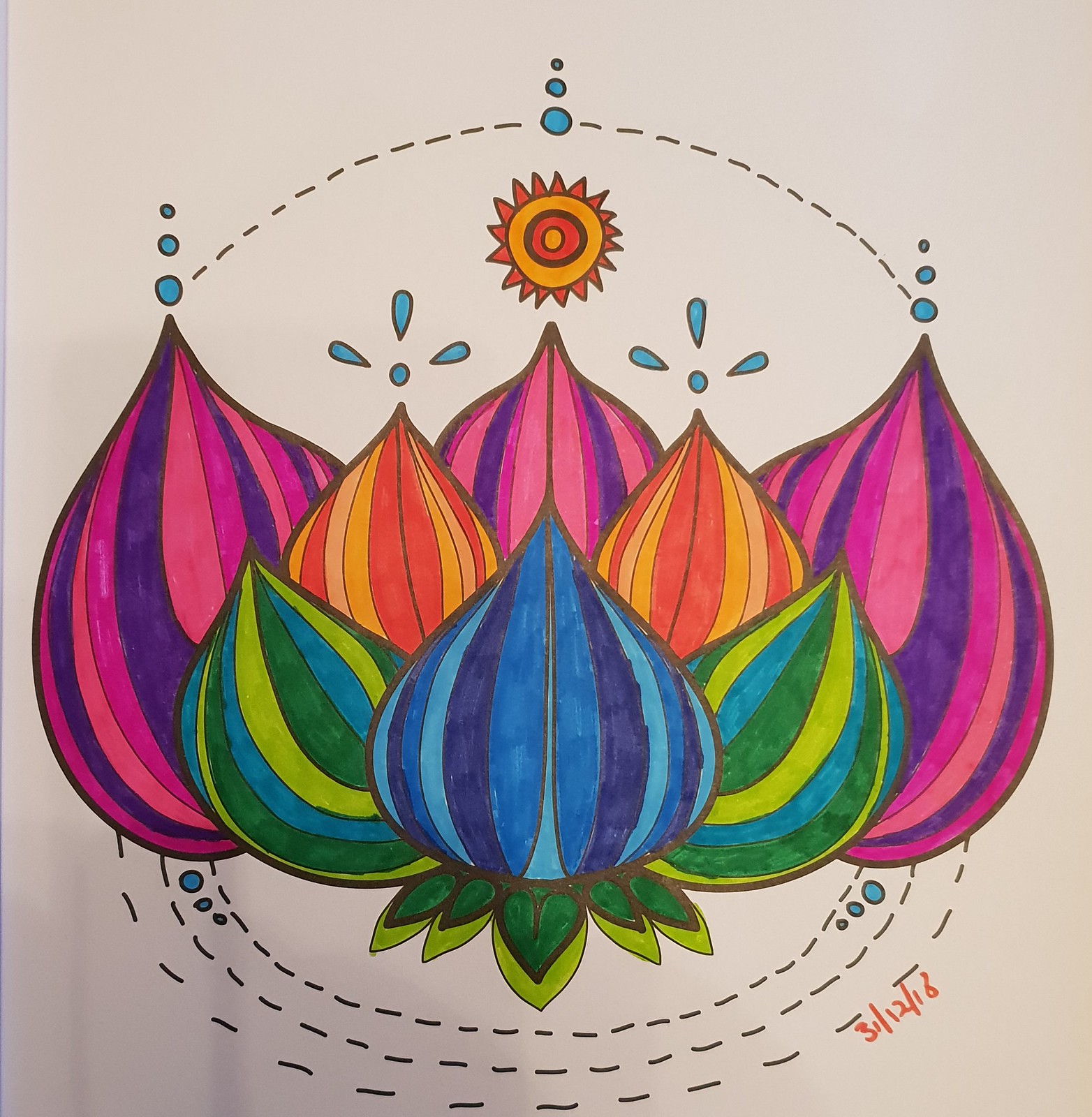This is a detailed drawing on light gray paper, rendered primarily with colored markers. The overall shape of the image is rectangular, with the longer sides on the left and right. Central to the artwork are multiple objects resembling flower buds or fruit, drawn and colored with vivid stripes. The buds have an elongated, bulbous shape akin to Hershey Kisses or garlic cloves, pointed upwards. 

From left to right, the buds exhibit a rich array of colors: the first is striped in purple, dark purple, and pink; the next is blue, transitioning into light green and dark green stripes; above this, there is an orange, yellow, and peach striped bud; and the final bud features stripes of light blue, dark blue, and turquoise. These colorful buds are surrounded by dotted lines: one dotted line arches above the topmost buds, while three dotted lines curve around the bottom buds. 

Distinctive orange handwritten marker text at the lower right reads "31-12-18." This sophisticated interplay of color and form is further enhanced by an intricate dot pattern and broken lines, encapsulating the dynamic and vibrant essence of the drawing.